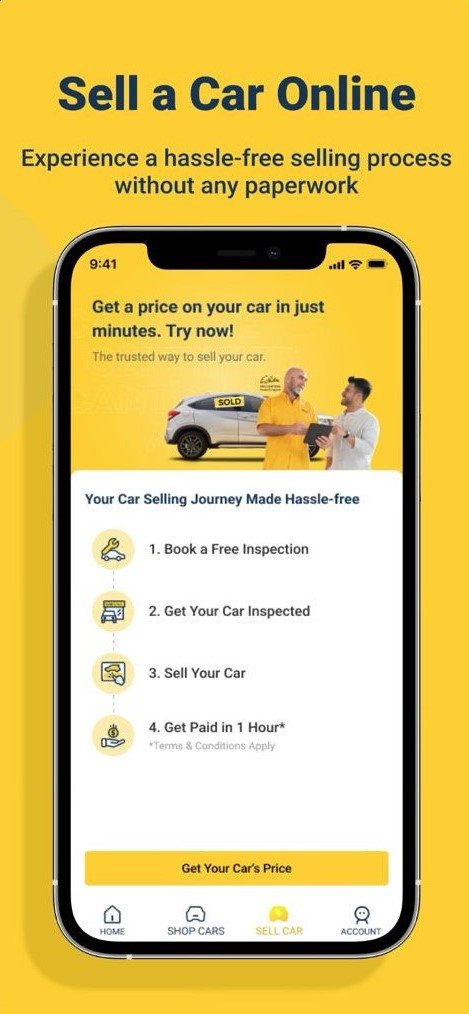**Detailed Descriptive Caption:**

The advertisement features a vibrant yellow background with key text and elements in striking blue and black font. The prominent headline reads "Sell a Car Online" in blue, highlighting the ease of experiencing a hassle-free selling process without any paperwork. Below it, an encouraging call-to-action states "Get a price on your car in just minutes. Try now." Encapsulating the trustworthiness of the service, the ad proclaims "The trusted way to sell your car," accompanied by a visual of a sold car, reinforcing the seamless nature of the selling journey.

The selling process is broken down into four straightforward steps:
1. Book a free inspection.
2. Get your car inspected.
3. Sell your car.
4. Get paid in one hour (*terms and conditions apply).

A detailed instruction box in bold black text, housed within a yellow rectangle, further emphasizes getting your car's price quickly and conveniently. Navigation options at the bottom in yellow, include "Home," "Shop Cars," "Sell Cars," and "Account," making the website easily accessible. Additionally, the ad displays a contact number, 941, ensuring direct communication for potential sellers.